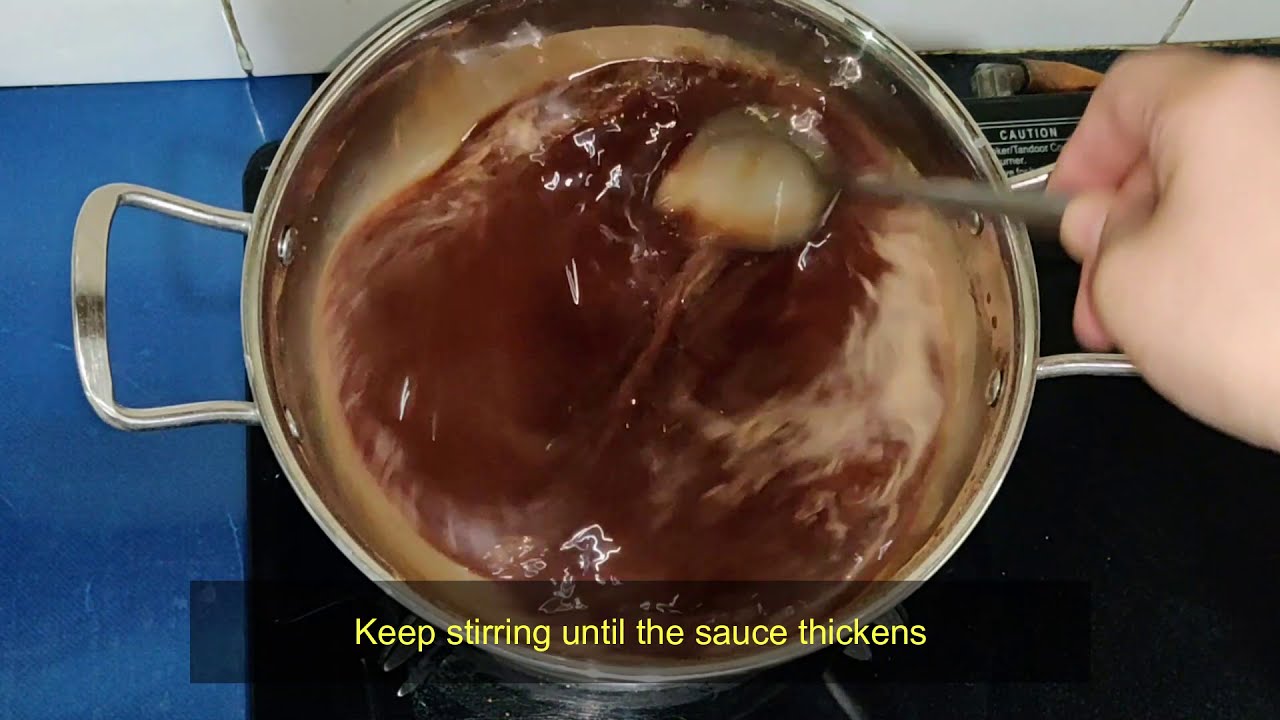The image depicts a detailed cooking scene from a video recipe, viewed from above. At the center of the photo is a stainless steel pot with U-shaped handles on both sides. Inside, a rich, brown sauce gently transitions from a light milk-chocolate color around the edges to a deeper, reddish-brown hue in the middle. A hand, likely of Caucasian descent, extends from the right, stirring the mixture with a silver spoon. This pot rests on a portable black cooktop, with a hint of a gas line visible at the back. Surrounding the cooktop, the surface appears to be a blue countertop, and the background reveals a white wall or tiled surface. At the bottom of the image, a black rectangle with yellow text reads, "Keep stirring until the sauce thickens."